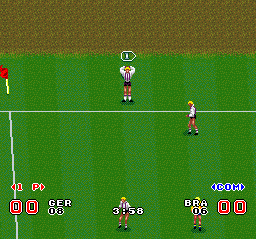This digital illustration or square screenshot captures the nostalgic essence of a 1980s vintage-style video game. The scene is set on a green playing field with distinct white lines, suggesting a sports setting, most likely a soccer game. A brown and light green textured wall forms the backdrop at the top edge of the image, adding to the retro aesthetic.

Four pixelated players are visible on the field, each adorned in white shirts, shorts, sneakers, and sporting yellow hair. The central player is positioned behind a vertical white line, arms raised, possibly indicating he's ready to receive or intercept the ball.

At the bottom of the image, numerical displays add context: on the left, "1P00" marks the player’s score, while "COM00" on the right indicates the computer’s score. Below the central player, a timer reads "358," tracking the game's progress. Over the player near the "COM00" indicator, the text "BRA06" appears, potentially denoting the team or player number.

The image employs a palette dominated by green, brown, yellow, white, blue, and black, emphasizing its charmingly simplistic and nostalgic video game design.